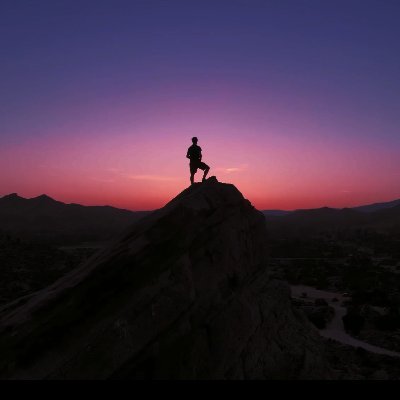A captivating photograph captures the silhouette of a man standing majestically atop a rugged mountain peak, right in the center of the image. He is poised with his left leg straight and his right knee bent, placing his foot on an elevated incline. His right arm is slightly bent at the elbow, adding to his relaxed yet triumphant stance. This breathtaking moment is set against a mesmerizing sunset, where the sky transitions from deep purple at the top, through shades of pink, to a soft blue near the horizon. The sun casts its final light behind distant mountain ranges. Below, a winding river snakes through the terrain on the right in an S-shape, glinting subtly in the fading light. Though the details of the foreground are shrouded in darkness, the sharp outlines of the man and the rocky outcrop he stands on convey a sense of solitude and accomplishment. The rocks, detailed with deep crevices and cracks, and the serene yet dramatic natural backdrop, emphasize the grandeur of the scene, making it a truly awe-inspiring snapshot of a moment in nature.